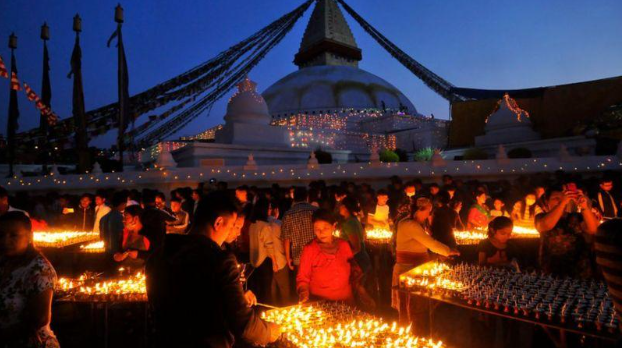The image depicts an outdoor religious ceremony likely in Nepal or India, showcasing an impressively well-lit scene. Hundreds of people, appearing to be of Asian or possibly Middle Eastern descent, are gathered around tables laden with candles, creating a sea of flickering lights that illuminate their faces, indicating a possibly festive or commemorative event. The backdrop features a grand domed building adorned with cascading ribbons or ropes, adding a festive and sacred atmosphere. The sky transitions from a dark blue on the left to a lighter shade on the right, enhancing the visibility of the myriad of bright colors worn by the attendees and emphasizing the end-of-day setting. Palm trees frame the scene, contributing to the authentic, cultural ambiance of the ceremony.